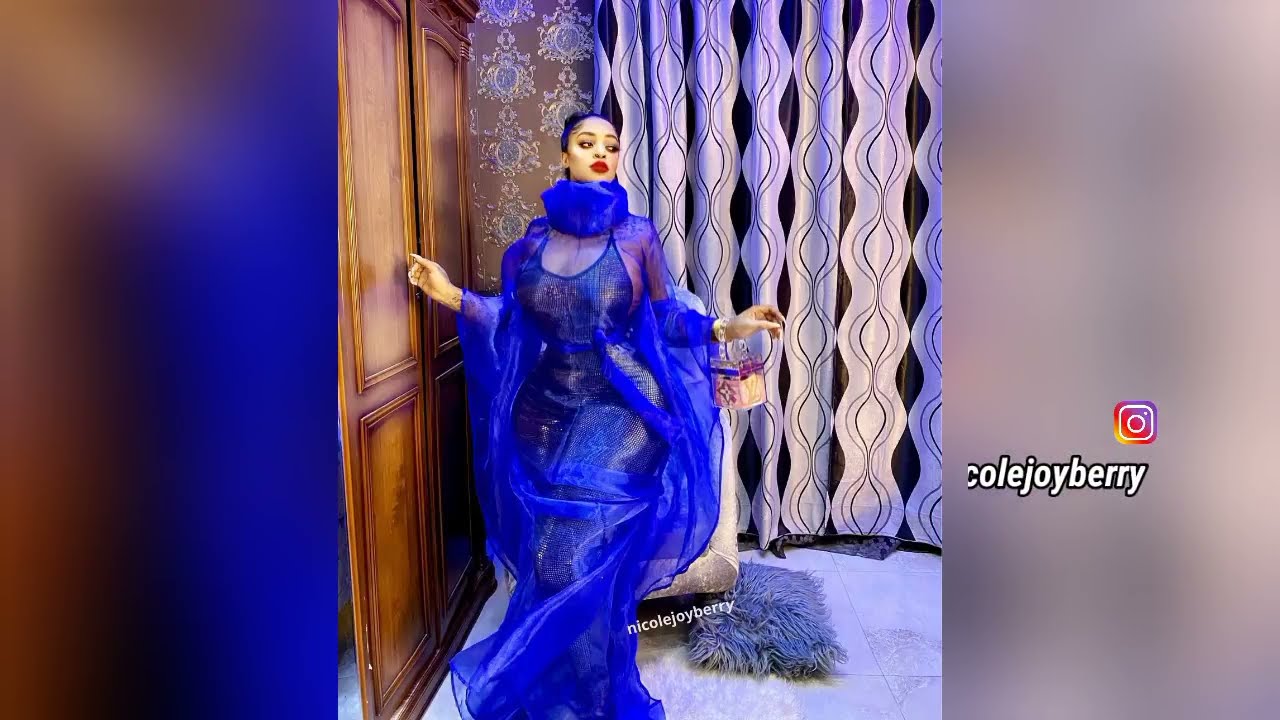In this detailed, horizontal rectangular image, the left and right 25% edges are heavily blurred, featuring a mix of bright blue and brown hues on the left and light gray and dark gray hues on the right. Dominating the in-focus center is a striking woman with darker skin, standing confidently with her arms slightly bent and hands dangling by her sides. She is dressed in an elegant, dramatic ensemble consisting of a lacy bright blue, flowy dress layered over a form-fitting, sleeveless black leather bodysuit. Her hair is black and pulled back, and she is adorned with vivid red lipstick and full makeup, including mascara and eyeliner. Her gaze is directed towards the bottom right of the image. 

Behind her hangs a black and white curtain with curved vertical lines, and she stands on a chic, shaggy white rug atop gray stone tiles. To her left, a set of brown cabinets is partially visible, while to her right, there is an Instagram logo above the username "Nicole Joy Berry" in white text. The same handle is repeated at the bottom of the image.